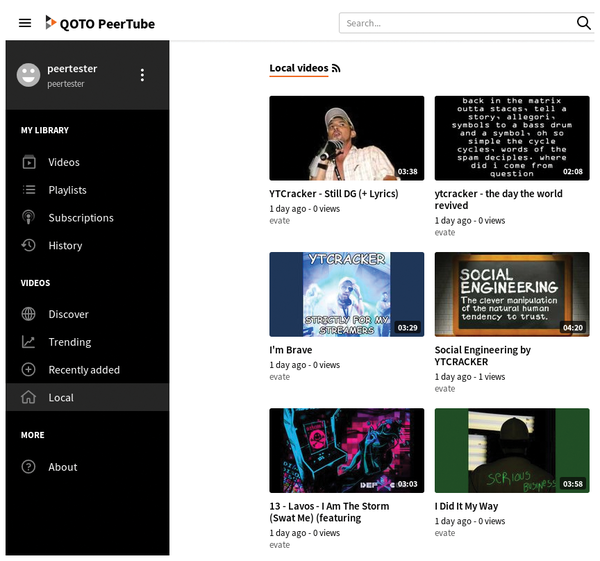The image is a screenshot of a user interface from a video viewing website named "QOTO PeerTube." In the top left corner, the text "QOTO" is written in all capital letters next to the PeerTube logo, which is an equilateral triangle pointing to the right. This triangle is composed of three smaller triangles: a black one at the top, a gray one at the bottom, and an orange one on the right, all touching at their edges.

On the left-hand side, there is a dark gray vertical sidebar labeled "peer tester" at the top with a small gray smiley face icon. Below this, the sidebar lists several options under the heading "My Library," including "Videos," "Playlists," "Subscriptions," and "History." Further down, under the section "Videos," are additional options such as "Discover," "Trending," "Recently Added," and "Local," with "Local" currently selected in gray. At the very bottom of the sidebar are options labeled "More" and "About."

On the right-hand side of the interface, the main section has a white background featuring a search bar at the very top. Below the search bar, "Local videos" is displayed in black text highlighted in orange. The main display area showcases six video thumbnails arranged in three rows of two each. The video titles from left to right, top to bottom, are as follows: "Why do you cracker still the G+ lyrics," "Why do you cracker the day the world revived," "I'm brave social engineering by YT cracker," "13 levels," "I am a storm SWAT me featuring," and "I did it my way."